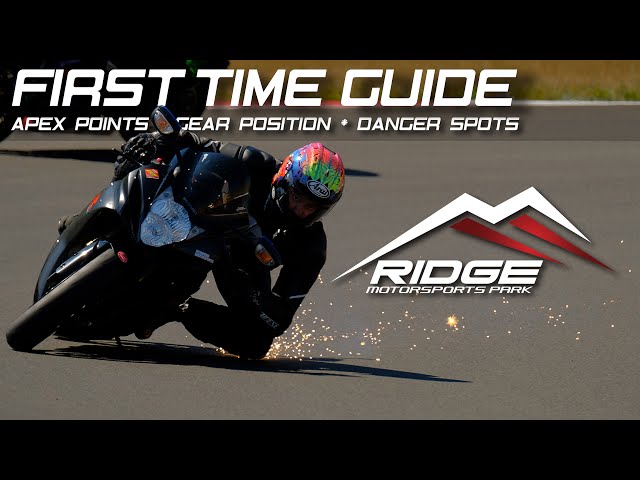This is a detailed and vivid photograph or video thumbnail captured during an intense motorcycle race. The image prominently features a motorcyclist in the midst of a sharp right turn, his knee skimming the asphalt and generating visible sparks due to the metal protectors. The rider's helmet is strikingly multicolored with a blend of white, green, pink, red, yellow, and blue. Dressed in a black racing jumpsuit, he maneuvers his black or dark blue motorcycle with precision and speed, his hands firmly gripping the handlebars.

The background of the scene reveals the gray racing track, juxtaposed with elements of dirt and greenery outside the track area, indicating natural surroundings. The photograph is framed with a black bar across the top and bottom, creating a horizontally rectangular shape.

At the top of the image, bold white text with a drop shadow reads "First Time Guide," followed by smaller text listing essential racing tips: "Apex Points, Gear Position, Danger Spots." A logo resembling white and red mountains is positioned to the right middle, accompanied by the text "Ridge Motorsports Park." This meticulously designed visual serves as an enticing advertisement or guide for enthusiasts of high-speed motorcycle racing.